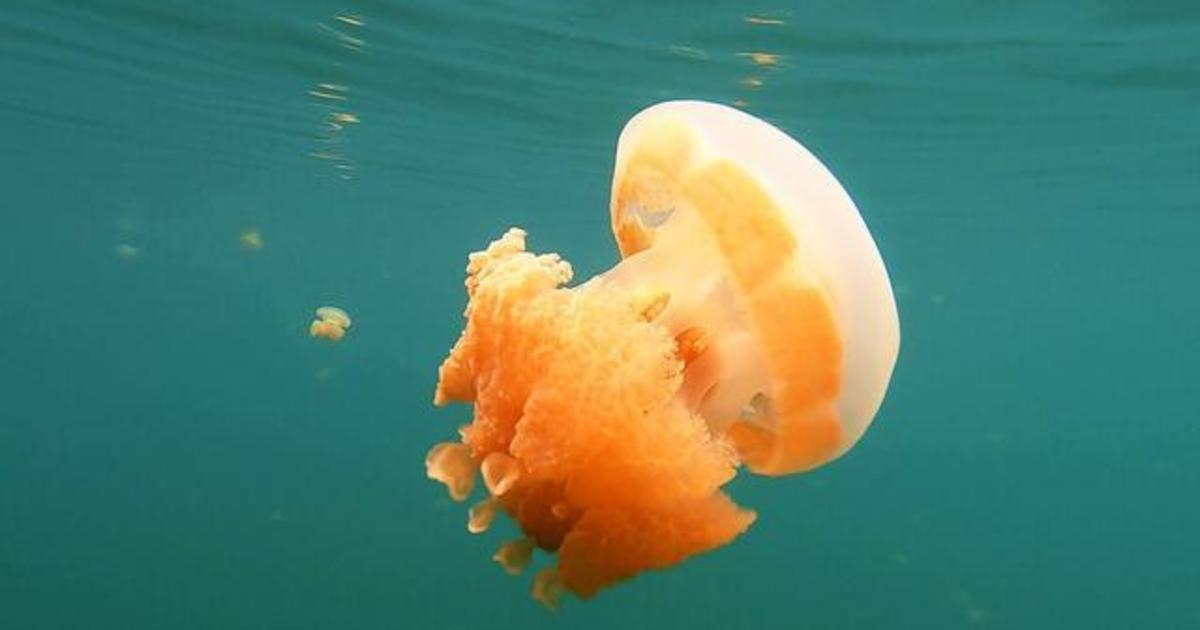The image is a horizontal rectangular photo taken underwater, featuring a clear, light turquoise background. At the center of the image is a close-up of a striking jellyfish, characterized by its translucent white, rounded cap resembling a mushroom. The cap transitions into an orangey color underneath, with sections appearing almost like coral. This jellyfish has a peculiar, almost balloon-like shape, and there are smaller fragments of the same material floating nearby. Supporting this scene, the water is dotted with additional jellyfish in the distance, and a few fish are faintly visible far off, contributing to the serene oceanic environment. This underwater photograph captures the ethereal beauty of these unusual, potentially stinging marine creatures.